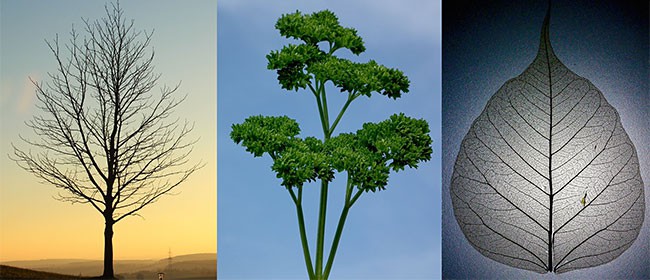The image is a horizontal strip featuring three distinct visuals. The first panel showcases a bare, deciduous tree silhouetted against a striking sunset backdrop. The sky transitions from a warm yellow glow near the horizon to a deeper blue higher up, with hints of a distant mountain range and possibly a tower accentuating the scene. The middle panel captures a sprig of parsley, its delicate stems and leaves sharply contrasted against a bright blue sky, intentionally mimicking the barren tree's form. The final panel on the right displays a highly detailed gray leaf, with its transparent quality allowing light to filter through and highlighting the intricate network of veins. The background is a gradient of light to dark blue, adding depth to the leaf's pale, almost powdery appearance. This composition ingeniously juxtaposes natural elements in a range of lighting conditions and perspectives, creating a cohesive and visually engaging narrative.